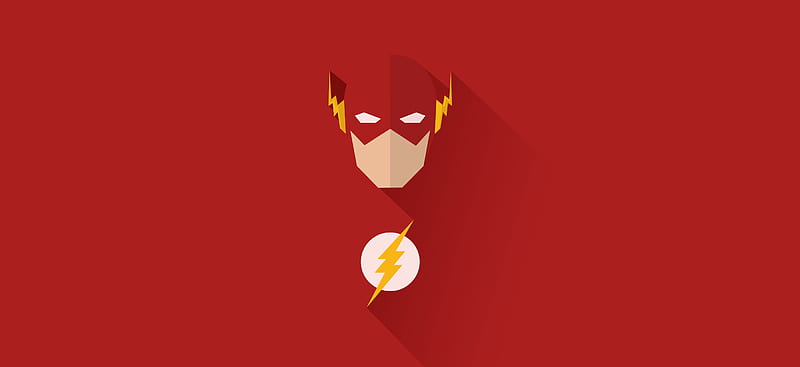The image depicts a minimalist design inspired by the superhero The Flash, set against a vivid cherry red background in a horizontal, rectangular format. Dominating the composition is the upper portion of a face adorned with The Flash's iconic red mask. This mask covers the head to the mid-face, leaving the flesh-colored lower half exposed and devoid of any features. The eye regions of the mask appear as white slits, giving a ghostly, enigmatic effect. Adjacent to the head are two prominent yellow lightning bolts, fashioned like ears, accentuating the dynamic nature of the character. Below the face, a circular white emblem with a striking yellow lightning bolt bisects the circle, reinforcing the superhero's emblematic iconography. The design's minimalist aesthetic and bold color scheme render it suitable for use as a wallpaper.